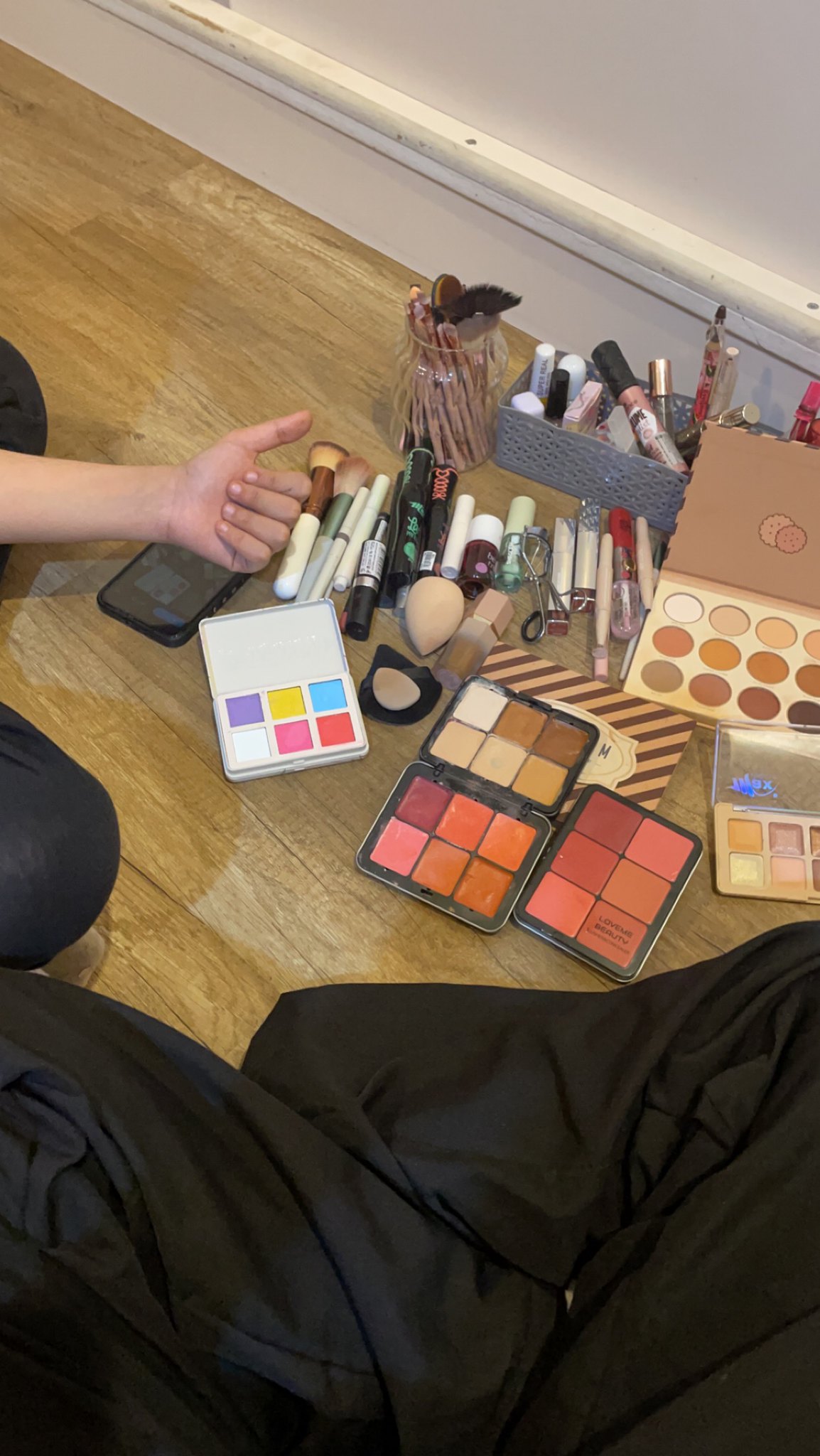In this overhead image, a person's forearm and hand are prominently visible. The person's fingers rest against the inner palm, with the thumb extended outward to the left. Below, a large collection of makeup items is arranged on the floor to the right. The setup includes rows of makeup brushes, a foundation sponge, and several makeup palettes.

One eyeshadow palette is white and contains vibrant colors, including purple, yellow, blue, white, pink, and red. Adjacent to it is another palette featuring various shades of brown, and below that, a palette displaying different shades of red and pink. The third palette nearby also has a selection of reds and pinks. To the right, there's another brown-colored palette offering a mix of red, brown, and lighter beige shades.

At the very bottom of the photograph, there appears to be the edge of a black blanket or sheet. Near the top, part of a white wall is visible. Additionally, a gray container sits in front, holding several makeup tubes with black and white lids. A circular container nearby holds makeup brushes with black tips.